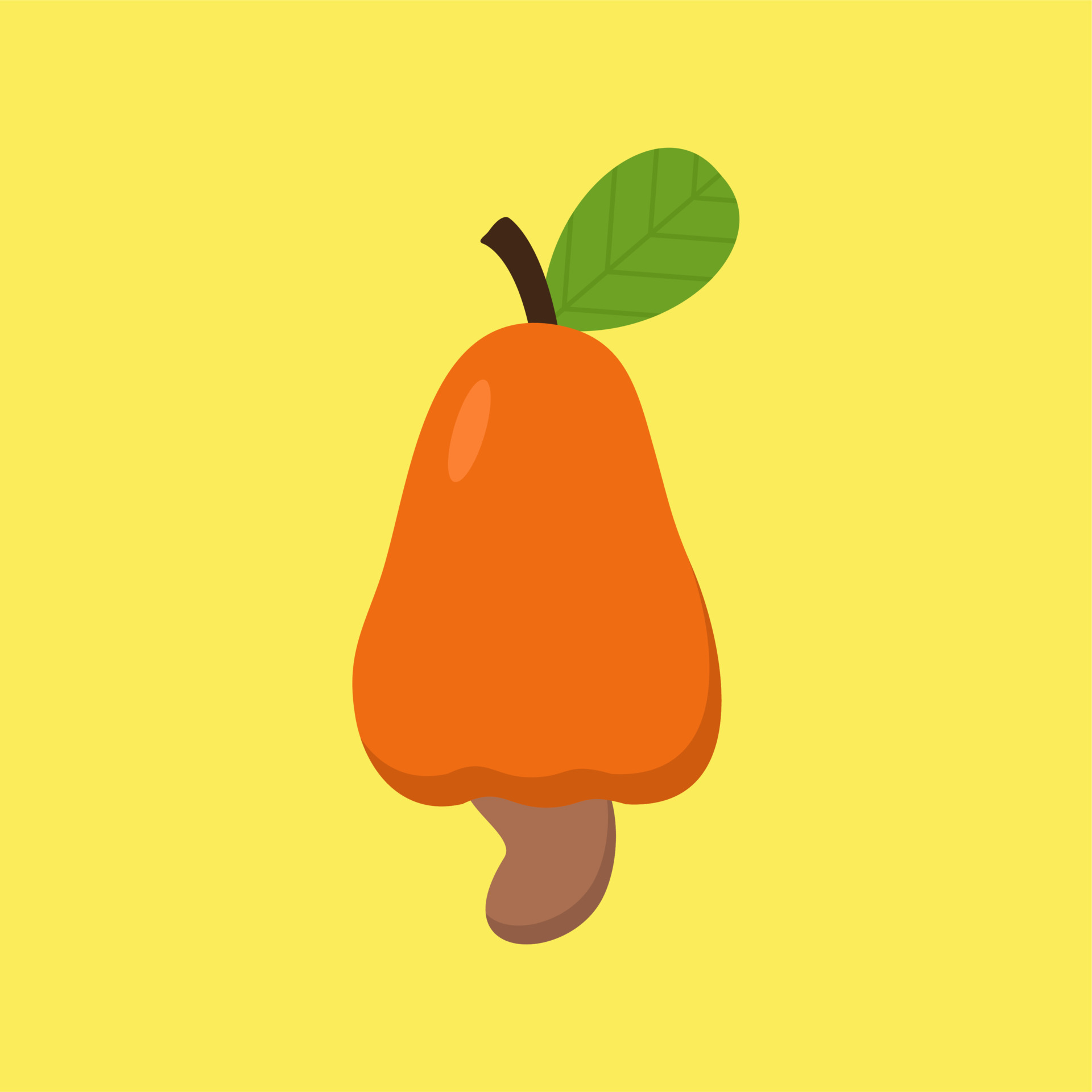Set against a vibrant yellow background, this image is a posterized pop art illustration in a square format, featuring an unconventional orange pear centrally positioned. The pear's distinctive bell shape is complemented by its vivid orange hue and subtle shadows on the upper left and lower sections, adding depth. The black, curved stem at the top tilts slightly to the left, crowned with a detailed, symmetrical green leaf directed towards the upper right corner, complete with intricate v-shaped veins and a central vertical line. Unusually, a brown, peanut-shaped protrusion extends from the bottom, adding a quirky twist to the composition.